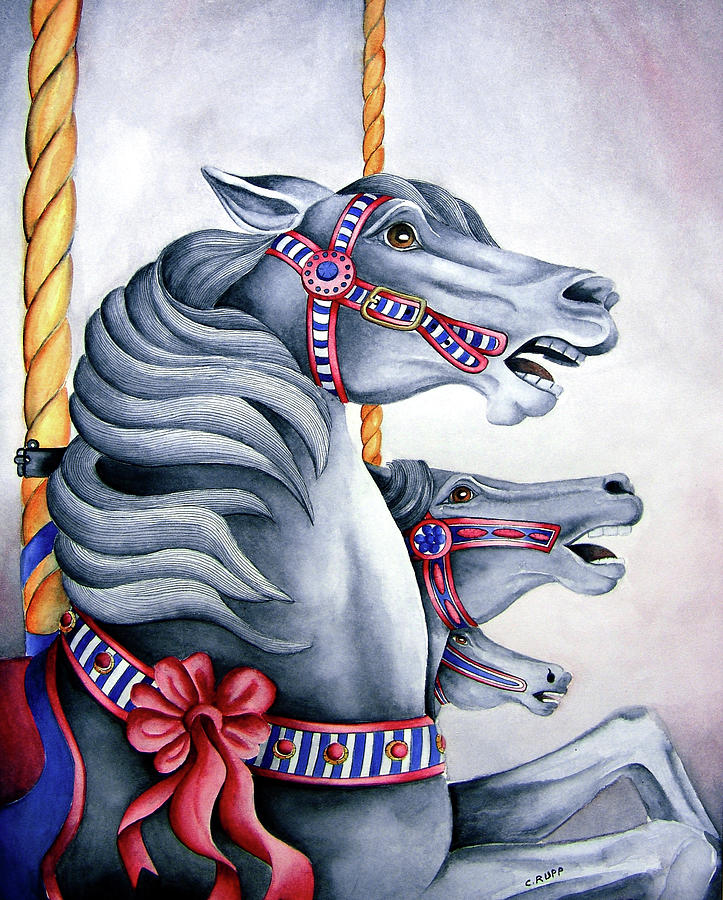This detailed illustration depicts a close-up view of three intricately drawn carousel horses against a bluish-purplish faded background. The primary horse, located at the forefront, boasts a grayish hue with its mouth open, revealing a sense of animated motion. This front horse also features a large red bow around its middle. All three horses are adorned with blue and white striped bridles, accented with red designs and flowers, contributing to a cohesive color scheme. 

The carousel poles from which the horses hang appear golden, imbuing the scene with a metallic glint that contrasts with the predominantly muted tones. Behind the primary horse, the faces of the other two horses are partially visible, each sharing a similar grayish coloration and open-mouthed expression. Their legs are all positioned to the right, suggesting a galloping motion. The artist’s initials, "C. Rupp," are subtly positioned at the bottom, marking the piece's authenticity. The illustration beautifully blends detailed craftsmanship with whimsical carousel imagery.